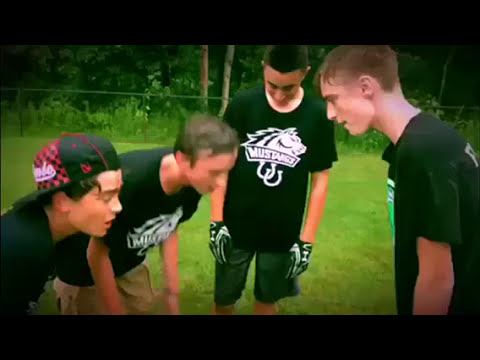In this image, four boys are standing on a lush green field, indicating they are part of a sports team. These boys appear to range in age from about 11 to 15 years old. They are wearing matching black t-shirts with a logo featuring a horse and horseshoes, and the word "Mustangs" prominently displayed, suggesting this is their team name. Despite minor variations, such as one boy wearing denim shorts and another in khaki bottoms, their uniforms are predominantly black and white. All the boys have short hair and appear sweaty, bent over as if catching their breath, with one boy on the left wearing a distinctive backwards red-and-black checkered cap with white text on it. In the background, there is a rope or chain-link fence, tall foliage including bushes, trees, and unmaintained grass, contributing to a natural, wooded area that frames the scene. There are no animals in the image, and the focus remains a close-up on the boys and their shared moment of rest and communication.